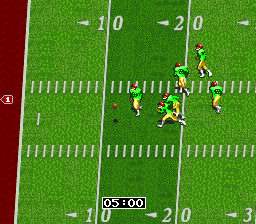This image appears to be a screen capture from an older version of a video game, likely Madden '93 on the Sega Genesis, depicting a football scene. The view shows a football field with distinct numerical markers at the 10 and 20-yard lines, displayed in white. Situated at the bottom of the screen is a black rectangular area with "05:00," indicating five minutes remaining on a timer. The field has a light green color with white lines crisscrossing it, and a dark green stripe running through the middle. A total of six players, dressed in neon green jerseys, red helmets, and yellow pants, are scattered across the field, seemingly engaged in a play. One player appears to be in the act of chasing or grabbing the football, possibly aiming to move left towards a potential touchdown. Near the goal line, marked by a red strip with white lines, there are various hashtags, adding to the game's classic visual layout.